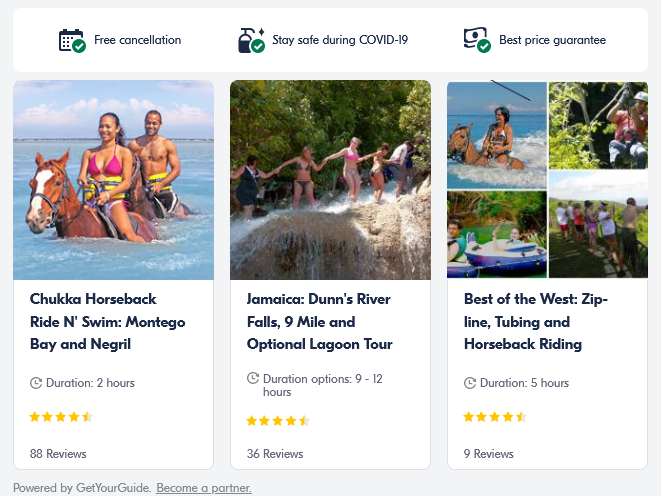This image is a detailed screenshot of a travel booking page, showcasing various features and options available to users. At the top left, there are three main location selections. Notably, the page includes several helpful icons and text:

- A "Free Cancellation" label with a calendar icon and a checkmark.
- A "Stay Safe for COVID-19" notice.
- A "Best Price Guarantee" badge with a dollar sign and a checkmark.

At the bottom left, there's a detailed section highlighting a specific activity:

- "Shoot, go horseback riding, swim on Tegel Bay" with a duration of two hours.
- Rated four stars based on 480 reviews.

Adjacent to it, on the right-hand side, there's another activity description:

- An image of people walking on Jamaica Falls, labeled "Jamaica Dunes or River Falls."
- Options for durations ranging from nine to 12 hours.
- The activity has a rating of approximately 4.3 stars based on 36 reviews.

Further to the right, there is another activity featuring:

- People riding on horseback, some near water, and others in a wooded area.
- Labeled "Best of the West Zip Line and Horseback Riding."
- Duration of five hours and a rating close to 4.25 stars from nine reviews.

At the bottom of the page, there is text in a grey background that reads:

- "Powered by Get Your Guide," with an underlying invitation to "Become a partner."

This comprehensive view gives users multiple travel and activity options, complete with descriptive captions, images, and user ratings to aid in their decision-making.